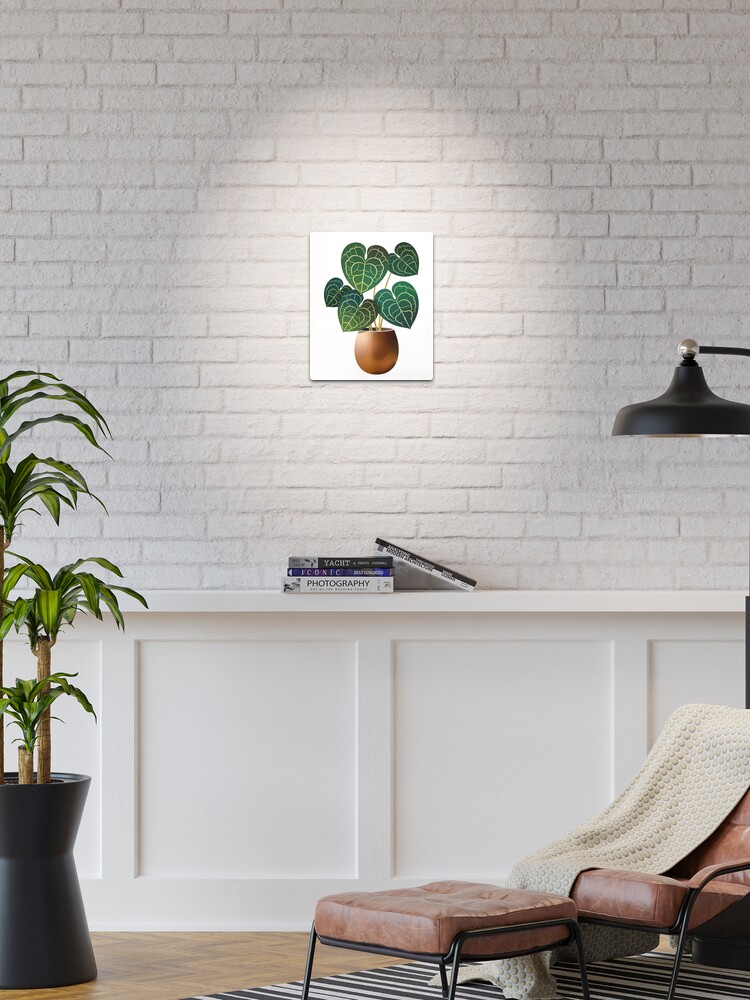A small, framed picture of a brown pot filled with vibrant green leaves hangs prominently on a white brick wall. The wall itself is an intricate design, with the upper three-quarters constructed from white brick, while the lower portion features an elegant wooden wainscoting with indented square patterns. A focused light shines directly on the picture, forming a circle of illumination around it. Below the white brick section runs a modest white ledge, housing a stack of three books, topped with an additional book leaning against them. Adding to the room's decor, a brown chair sits in the foreground next to a tall plant with a black base, resembling mini palm trees. The room's flooring is brown, complemented by a striped white carpet that lies beneath the chair, providing a cozy and stylish touch.